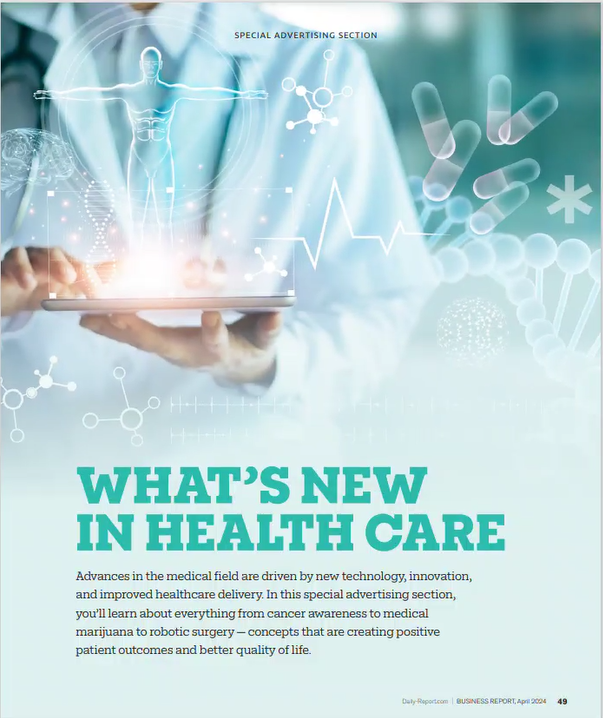The advertisement visually showcases the latest advancements in healthcare. Dominating the top portion is a figure in a white lab coat, holding a tablet with their left hand while interacting with it using their right index finger, which illuminates a bright light at the touchpoint. Emerging from the tablet, there is a holographic display depicting a human figure in a T-pose, symbolic of health and vitality, surrounded by various medical images. These images include translucent pills, an EKG readout, a stylized atomic or molecular structure, a double helix DNA strand, and a brain. The main text, displayed in bold, bright blue letters, reads "WHAT'S NEW IN HEALTHCARE," followed by a detailed description highlighting how recent technological innovations and improvements in healthcare delivery are driving advances in the medical field. It mentions topics such as cancer awareness, medical marijuana, and robotic surgery, all contributing to positive patient outcomes and better quality of life. This advertisement appears on page 49 of the business report.